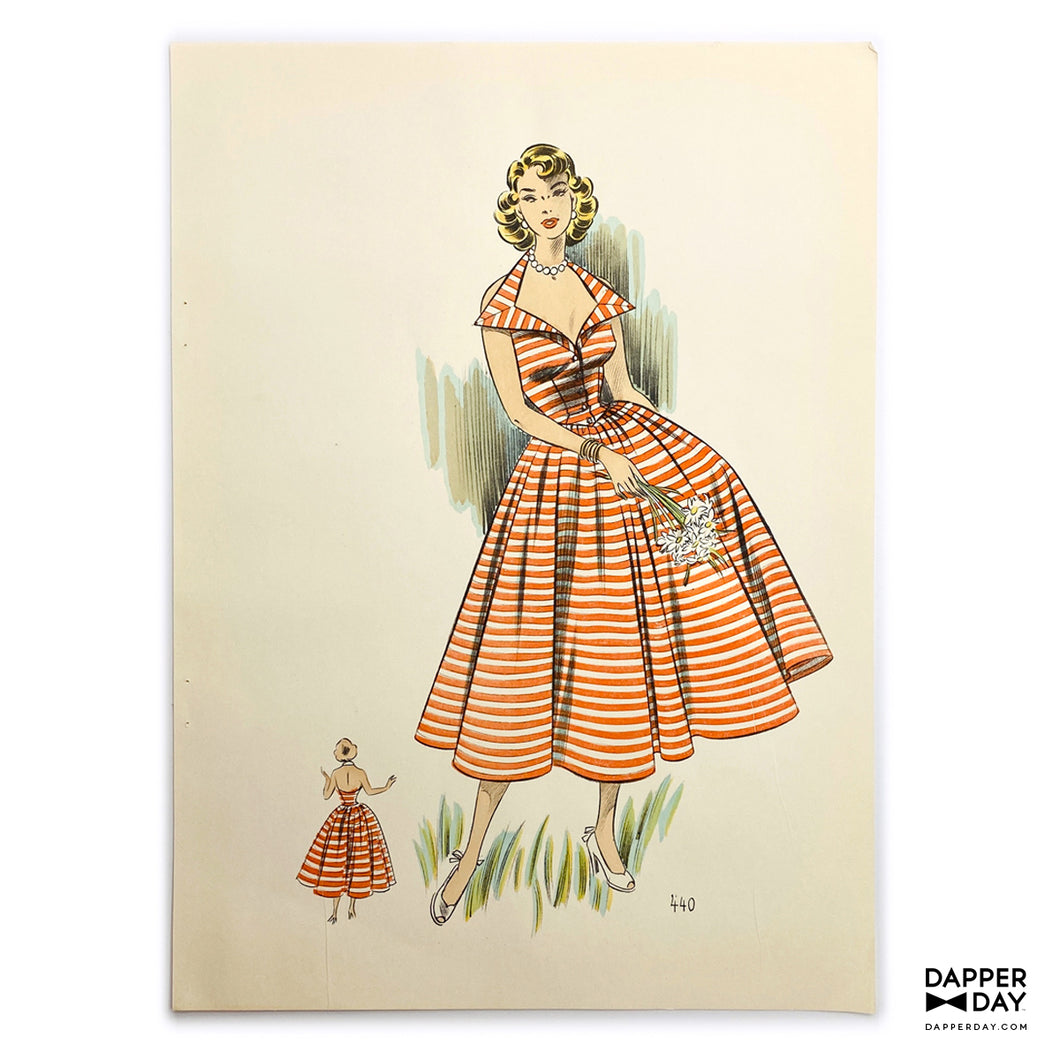This is a detailed vintage fashion illustration of a woman with shoulder-length, permed, curly blonde hair and white, open-toed high-heeled shoes. She is wearing a striking red and white horizontal striped dress, evocative of the 60s style. The dress features a wide-lapel, open V-neck collar that flares out in a diamond shape, and is sleeveless with a fitted bodice and a long skirt that falls to mid-calf. Her elegant ensemble is accessorized with a pearl necklace consisting of about six or seven pearls, and she holds a bouquet of white flowers in her right hand, adding a summery, casual touch to her appearance. 

The creamy-colored paper background of the illustration is decorated with dashed lines resembling blades of grass extending from behind her feet and torso. To the bottom left, a smaller illustration depicts the back view of the dress, highlighting its backless design. This lithograph includes the pattern number 440 and features a logo on the white exterior of the image that reads "Dapper Day" with a little bowtie, associating it with DapperDay.com.